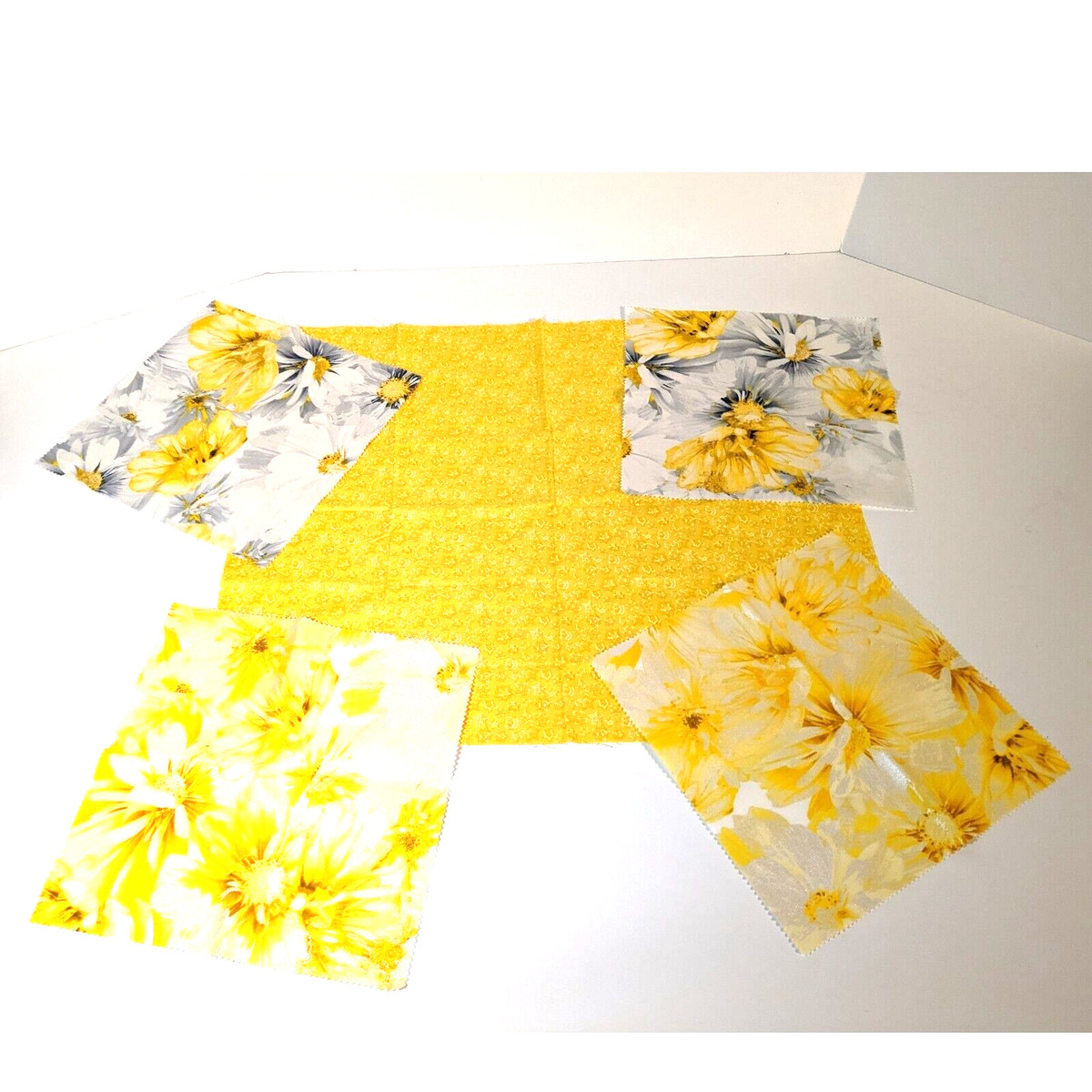This photograph showcases a selection of fabric squares meticulously arranged on a white surface in a brightly lit, white-walled room. The central piece is a large, vibrant yellow square, approximately two feet by two feet, displaying a subtle, textured floral design. Resting on the corners of this prominent yellow piece are four smaller fabric squares, each a quarter of its size. These smaller squares feature various floral patterns in a coordinating color palette of yellows, oranges, grays, and whites.

The two upper squares depict flowers with white and gray petals, highlighted with bright yellow centers akin to daisies. The bottom left square is predominantly yellow, bursting with bright floral designs that stand out more intensely, possibly due to the lighting. The bottom right square also features yellow flowers, blending seamlessly with the other fabrics. The cohesive color scheme and careful positioning suggest these are fabric swatches intended for a quilting project or similar craft, offering a harmonious visual and tactile preview of the materials.